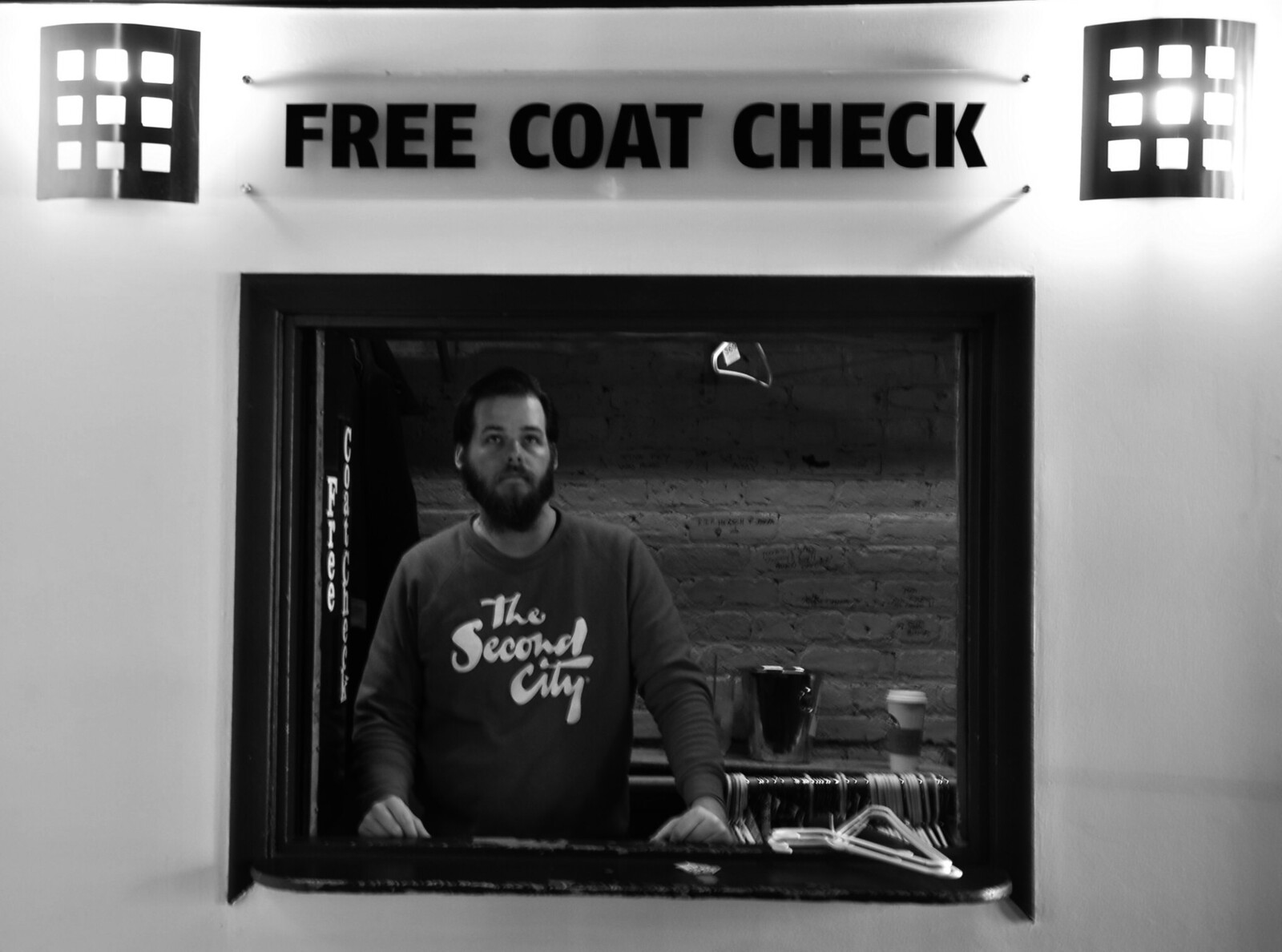This black and white image appears to be taken inside the lobby of a theater or similar event space. In the upper left and right corners, there are distinctive lighting fixtures resembling black steel grates with three-by-three checkerboard patterns of white squares. Centered between these fixtures is an illuminated sign with black text reading "Free Coat Check." Below the sign, there is a service window bordered in black, creating a frame-like effect. 

Inside the window, an attendant stands ready to assist. The attendant, a man with a beard and mustache, wears a dark long-sleeve shirt adorned with the text "The Second City" in a font that appears spray-painted. To his left are several plastic hangers and a Starbucks cup, placed on the ledge of the window. He is stationed against a backdrop of white brick wall, suggesting that the building might have a repurposed industrial or warehouse design. The overall scene captures the organized and ready atmosphere of the coat check service area.